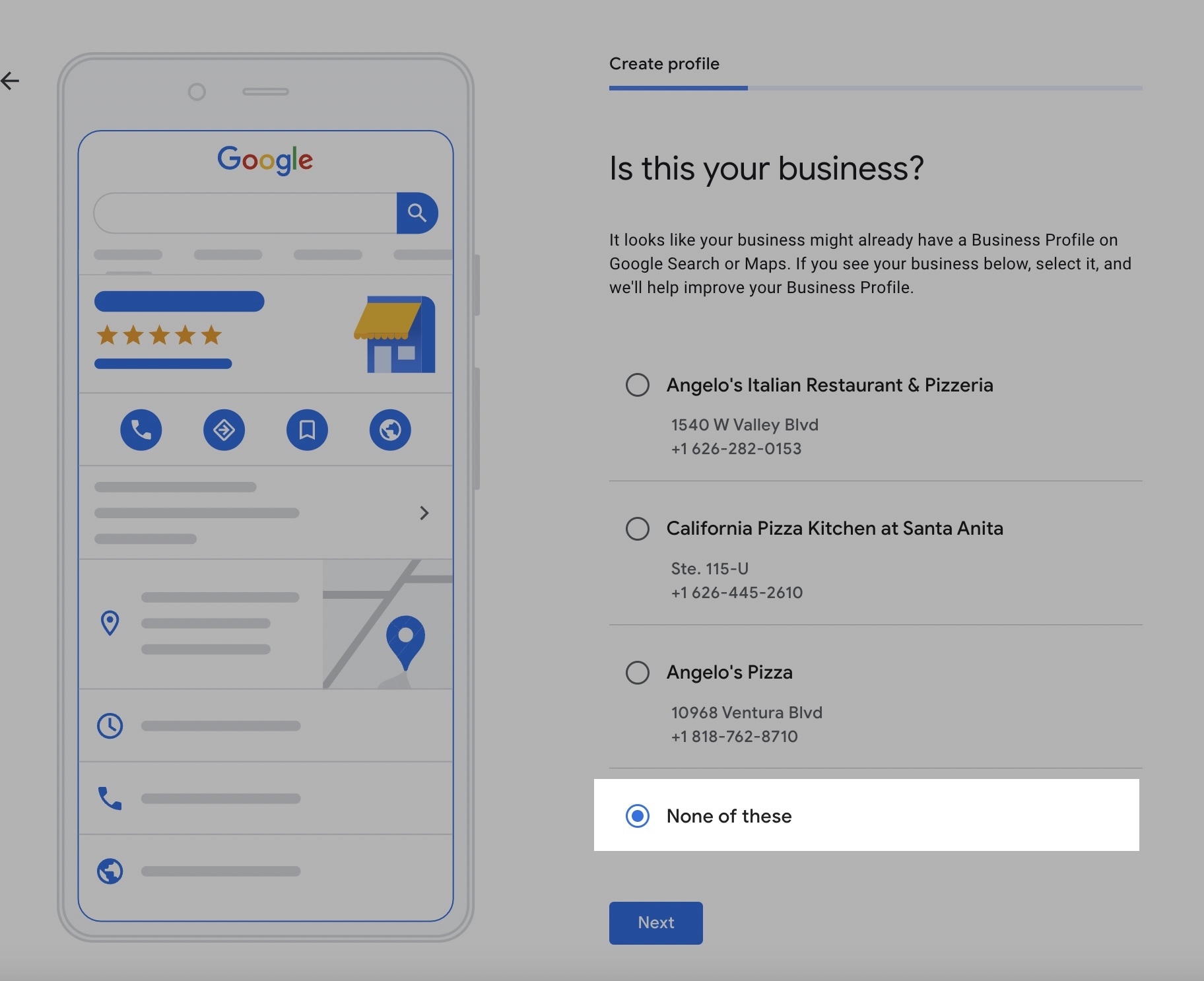Here is a detailed and cleaned-up caption:

---

This screenshot displays a step-by-step guide on how to create a Google Business Profile. The background of the image is a muted gray, highlighting the instructional content prominently. On the left side of the screen, there is a depiction of a smartphone showcasing a Google Business Page demo. At the top of this phone screen, it reads "Google" above a search bar, illustrating how the business profile will appear in Google Search results.

The profile demonstration includes various icons representing features such as star ratings, call, directions, save, and website links. Below these icons, there are additional symbols indicating how the business's address and operating hours will be displayed.

On the right side of the image, a header at the top reads "Create Profile," accompanied by a horizontal progress bar indicating the status of the setup process. The progress bar's initial segment is shaded in blue, signifying the first step is in progress. Below this bar, the text prompts users with, "Is this your business?" and continues to explain, "It looks like your business might already have a business profile on Google Search or Maps. If you see your business below, select it and we'll help improve your business profile."

Following this prompt, there are four business listings provided as options:
1. **Angelo's Italian Restaurant and Pizzeria**
   - Address: 1540 West Valley Boulevard
   - Phone: +1 626-282-0153
2. **California Pizza Kitchen at Santa Anita**
   - Address: Suite E115
   - Phone: +1 626-445-2610
3. **Angelo's Pizza**
   - Address: 10968 Ventura Boulevard
   - Phone: +1 818-762-8710
4. **None of these**
   - This option is highlighted in white.

At the bottom of this section is a blue button labeled "Next," indicating the continuation to the next step in the profile creation process.

---